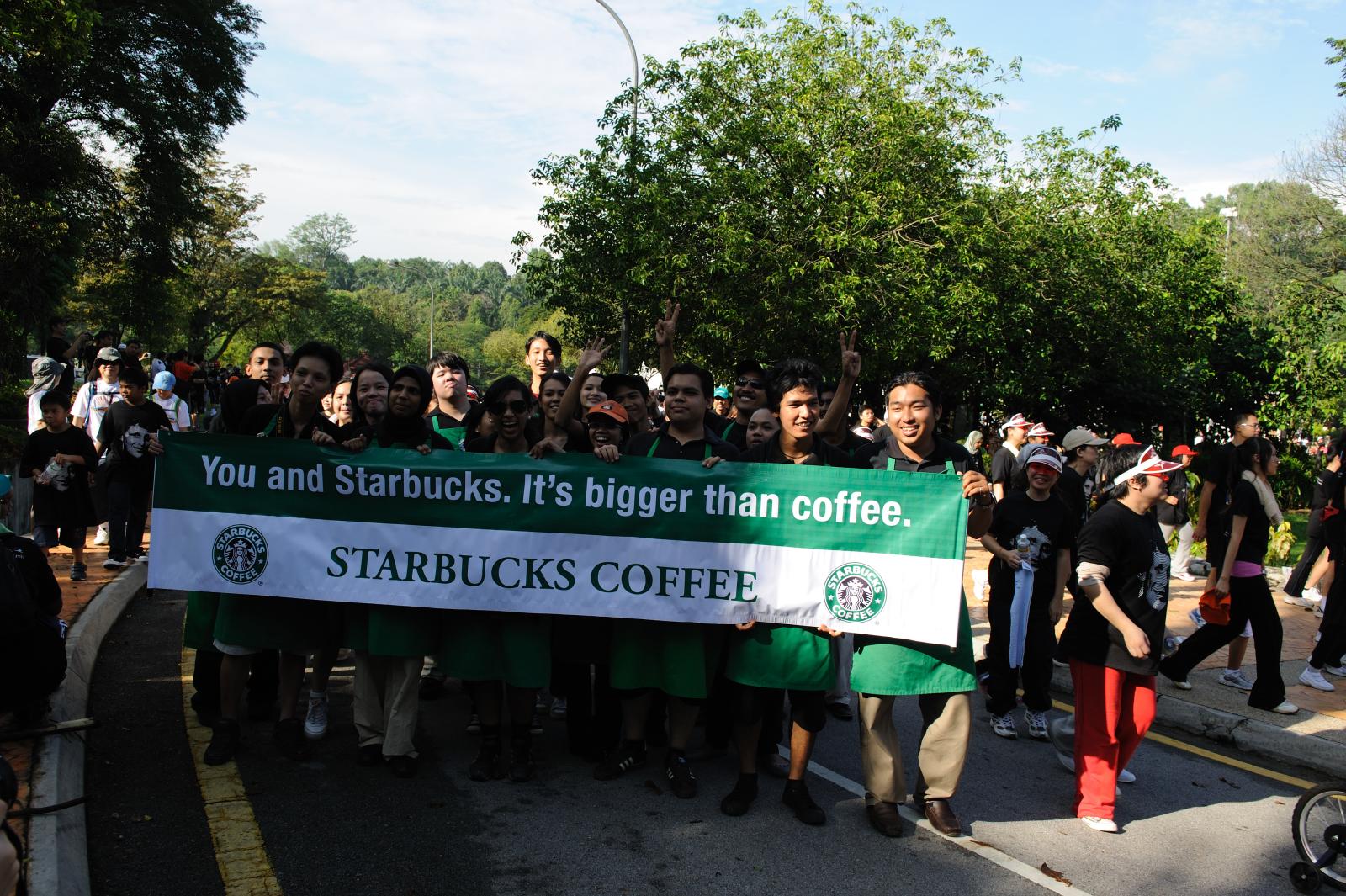In the image, an energetic group of mostly young people—who appear to be of Asian or Indian descent—is marching down a narrow, two-lane street under a bright blue sky dotted with white clouds. The scene is vibrant and filled with sunlight, casting striking shadows and illuminating the faces of the participants. Surrounding the marchers are verdant trees lining the street and sidewalks populated with onlookers.

At the forefront, a noticeable contingent of marchers, some clad in Starbucks uniforms consisting of black tops, chino pants, and iconic green aprons, is carrying a striking green and white banner. The banner prominently displays the phrases "You Win Starbucks" in white on the green upper part and "Starbucks Coffee" in green on the white lower part. Flanking these words on both ends of the banner are the recognizable Starbucks logos.

Among the front-row participants, one individual in the center stands out with khaki pants and another to their right sports a red and white visor emblazoned with a face design, red pants, and white shoes. The size of the crowd suggests a significant gathering, possibly a rally or parade, aiming to make a statement about Starbucks' impact or branding. The natural backdrop and the multicultural vibe of the group add a lively and diverse essence to the scene.